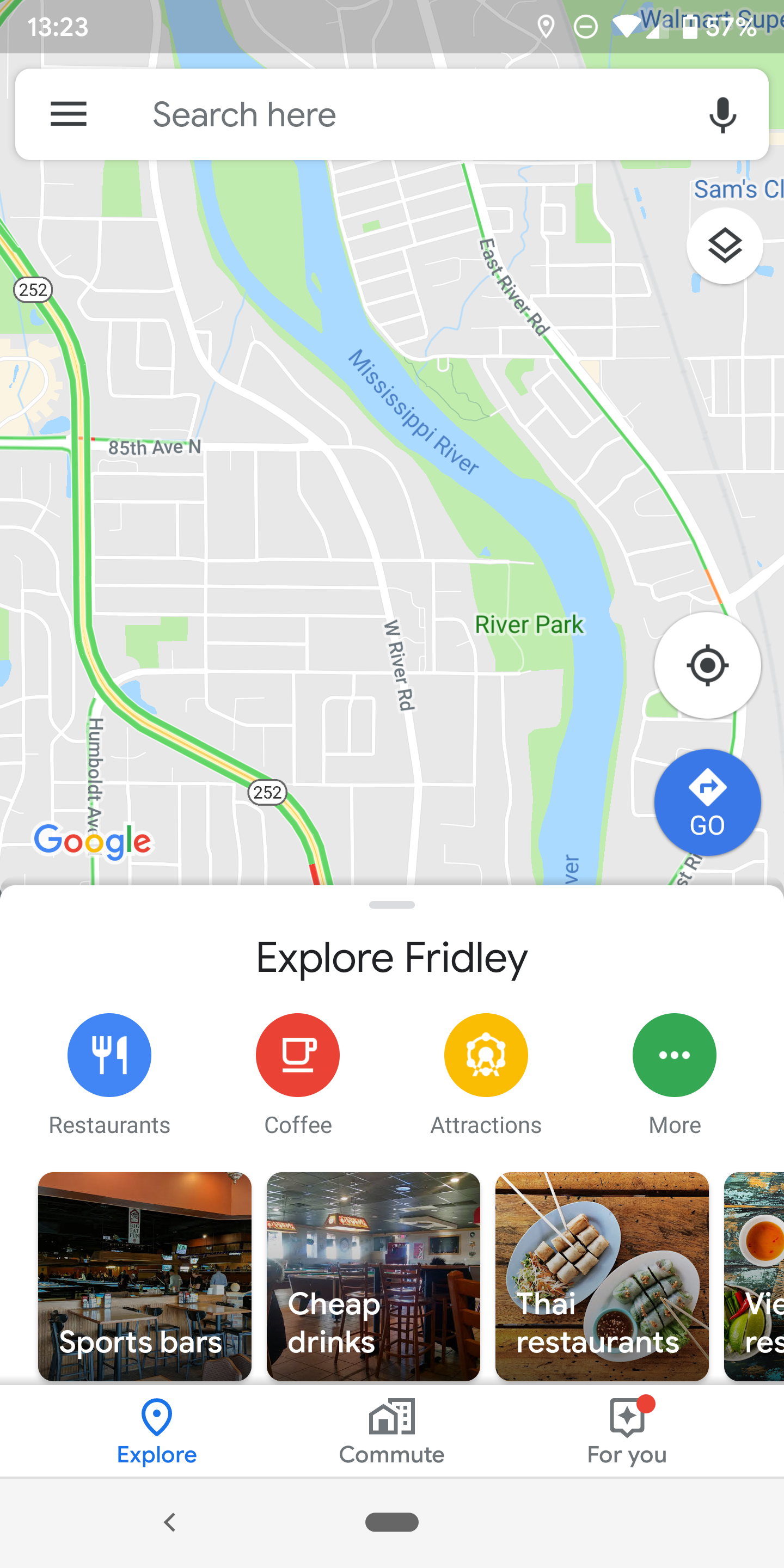The screenshot depicts a cell phone screen with various elements. The time "13:23" is displayed in the top left corner, while the top right corner shows icons for wireless connection and battery status. Below these, a search bar prompts "search here."

Dominating the screen is a map, identifying key locations such as the Mississippi River, River Park, East River Road, and 85th Avenue North. Beneath the map, the phrase "Explore Freely" appears, followed by four categorized icons:

1. A blue circle with a white fork and spoon, labeled "Restaurants."
2. A red circle with a white coffee cup, labeled "Coffee."
3. A yellow circle featuring a Ferris wheel, labeled "Attractions."
4. A green circle with three white dots, labeled "More."

Below these icons are four photos, three fully visible and one partially cropped on the far right:

1. The first photo on the left shows the interior of a sports bar, featuring tables, chairs, a bar area, and some patrons in the background. It is labeled "Sports Bars" with a blue pin and the word "Explore" in blue text underneath.
2. The second photo depicts the interior of a bar area with high stools and chairs, labeled "Cheap Drinks."
3. The third photo showcases plates of Asian food, labeled "Thai Restaurants."